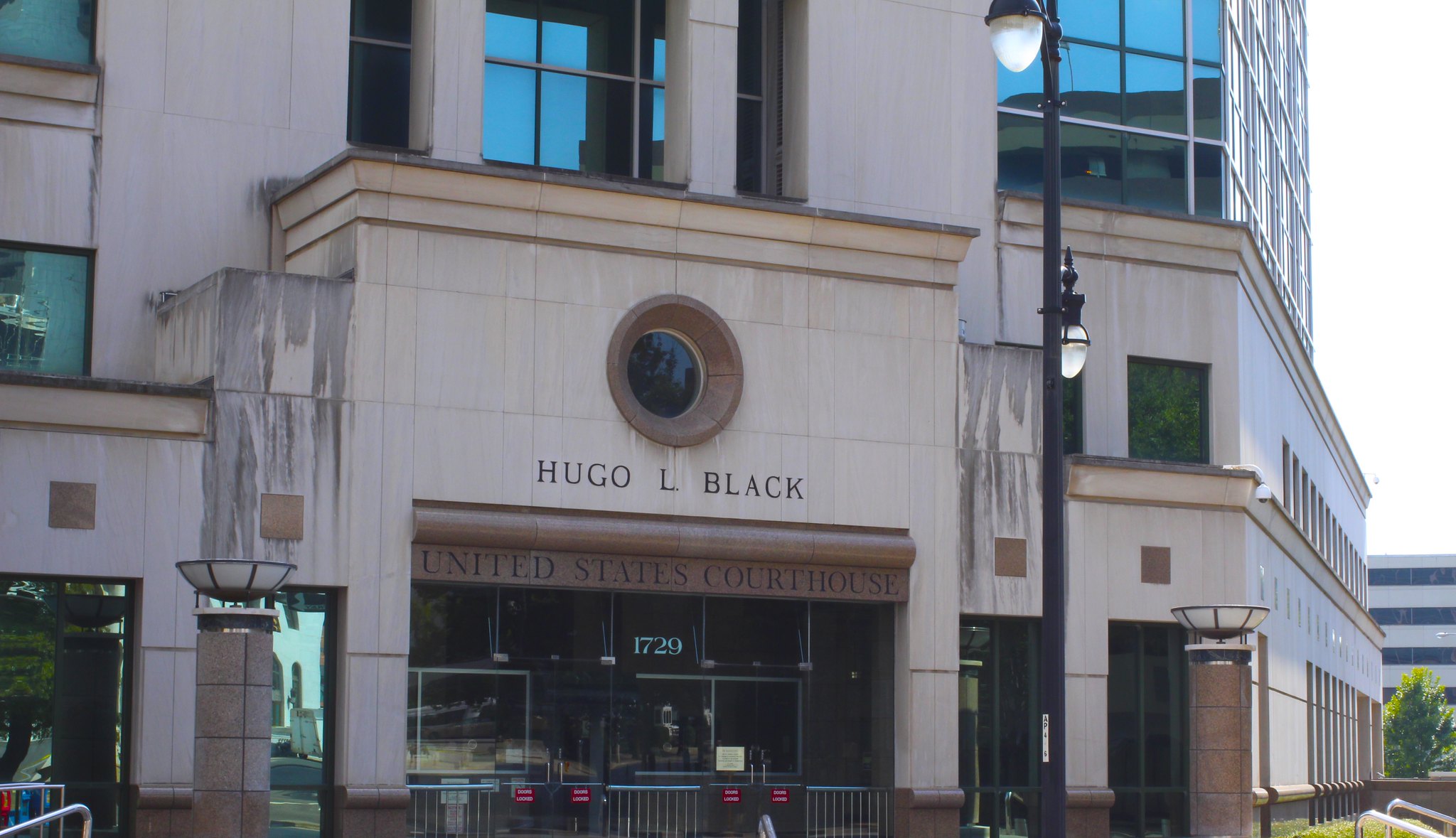This color photograph, oriented in landscape mode, captures a detailed front view of the multi-story Hugo L. Black United States Courthouse in Birmingham, Alabama. The building's façade, made of light brown square stones with dark and light concrete elements, is reflected beautifully in its windows, some of which mirror the clear blue sky and patches of green from nearby surroundings. Prominently featured in the center is a large, wide glass gate with "United States Courthouse" inscribed above it, and further above, "Hugo L. Black" is etched into the stone, beneath a distinct circular design with flared dark brown trim. The image, taken from across the street, includes street-level details such as grass patches, a touch of greenery, and several lampposts. Notably, a black lamppost with acorn-shaped lighting fixtures stands just right of the center. The courthouse address, 1729, is also visible, emphasizing its stately presence and architectural realism.